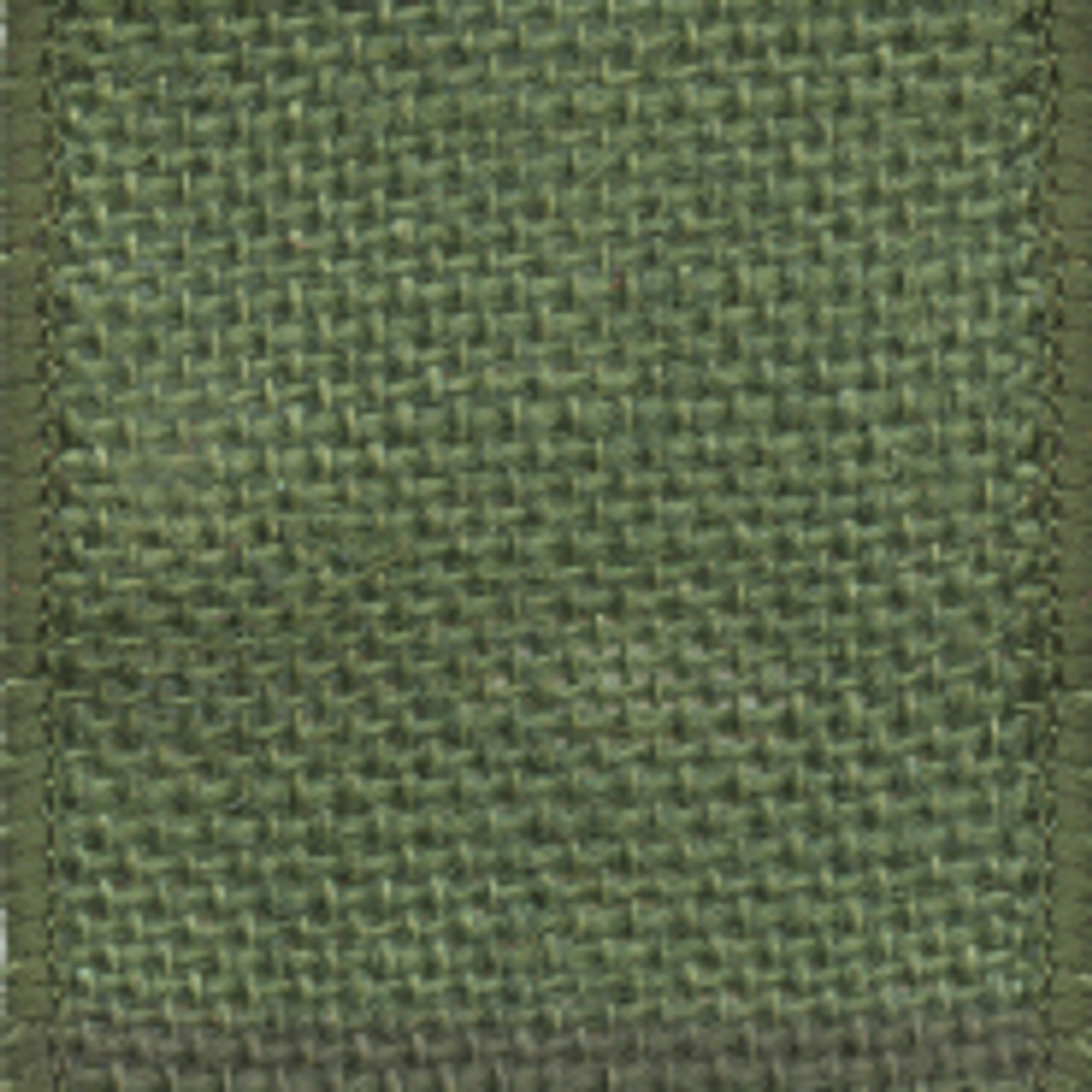The image features an extremely zoomed-in view of a textile, revealing the intricate interlinked threads that form a dense, net-like pattern. The fabric, possibly a piece of clothing, blanket, or another knitted or crocheted item, showcases a square section with a border visible on three sides. The predominant colors are muted shades of gray with subtle hints of blue, some specks of white, and perhaps traces of black, giving a slightly varied yet cohesive appearance. The texture and tight weave suggest it could be anything from a cable-knit sweater to a scarf or even a placemat. Despite the item taking up the entirety of the image and appearing slightly crooked, it maintains a mostly symmetrical shape. The close-up nature of the photograph makes it difficult to discern the exact type of textile, but the detailed view of the yarn and stitching highlights the craftsmanship, resembling a finely woven, monochromatic basket pattern.